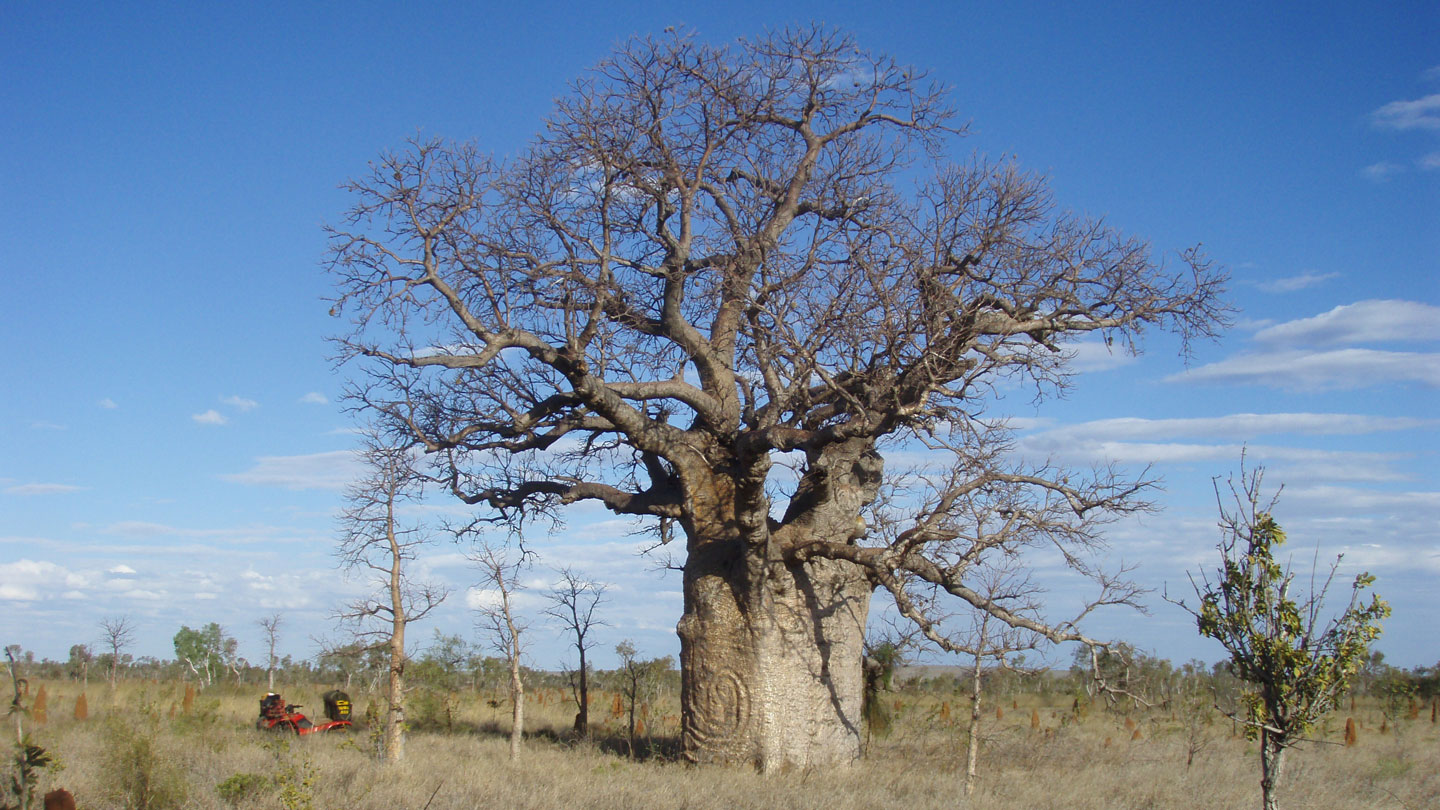The image captures a majestic, ancient tree in a savannah grassland, characterized by its extremely wide and thick trunk, which is wider than typical trees. The tree's trunk splits into two primary branches and then further into numerous smaller branches that spread broadly, almost as wide as the tree is tall. This striking tree, with its grayish, gnarled appearance, stands bare, devoid of leaves, giving it a stark, almost eerie look against the vivid blue sky. Around it, the grass appears dry and brown, suggesting a drought or lack of recent rainfall. Flanking the large tree are several smaller, equally barren trees, with the exception of one on the right that has some green leaves. Prominently, there is a four-wheeled red and black vehicle parked 15 to 20 feet away on the grassy plain, offering a sense of scale to the scene. Additionally, there is a crude drawing of a snake carved into the trunk, along with a protrusion resembling a nose, adding a unique, almost human-like quality to the tree. This serene daytime scene lacks any visible signs of animal life, emphasizing the tree's solitary dominance in this vast, open landscape.